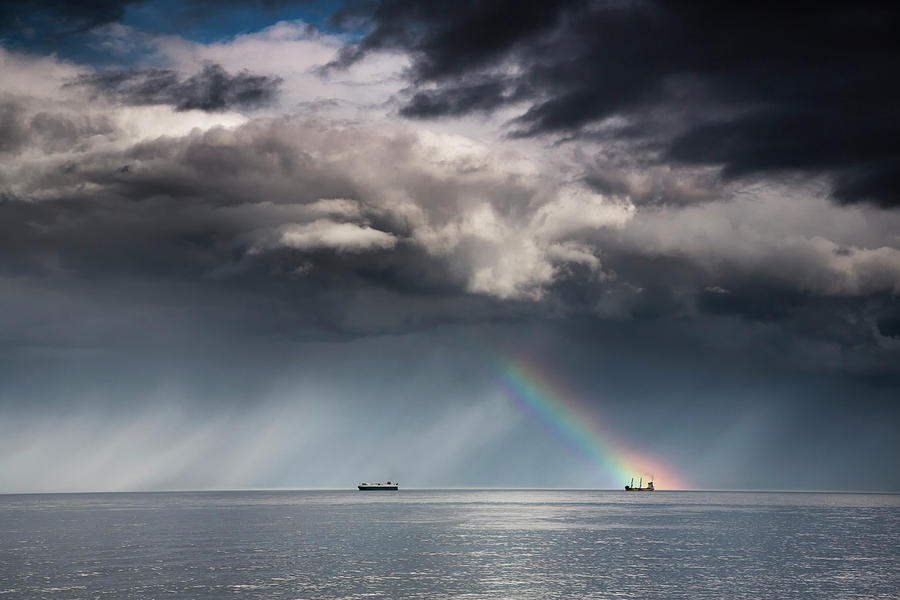This photograph captures a strikingly dramatic scene over a calm, slate-gray ocean. The sky above is filled with an array of tumultuous storm clouds, ranging from stark white to ominous black, with streaks of rain or sunlight breaking through in the distance. Dominating the right side of the image, a vibrant rainbow arcs down from a cloud to touch the water, its colors vividly transitioning from purple to red. Notably, the tip of this rainbow appears to converge upon a distant ship, possibly a sailboat with its tall masts, creating a captivating focal point. Another ship, likely a cargo vessel, is positioned closer to the center while traveling across the lower part of the frame. The overall scene is a mesmerizing interplay of natural elements, highlighting both the serene flatness of the ocean and the dramatic, contrasting sky above.